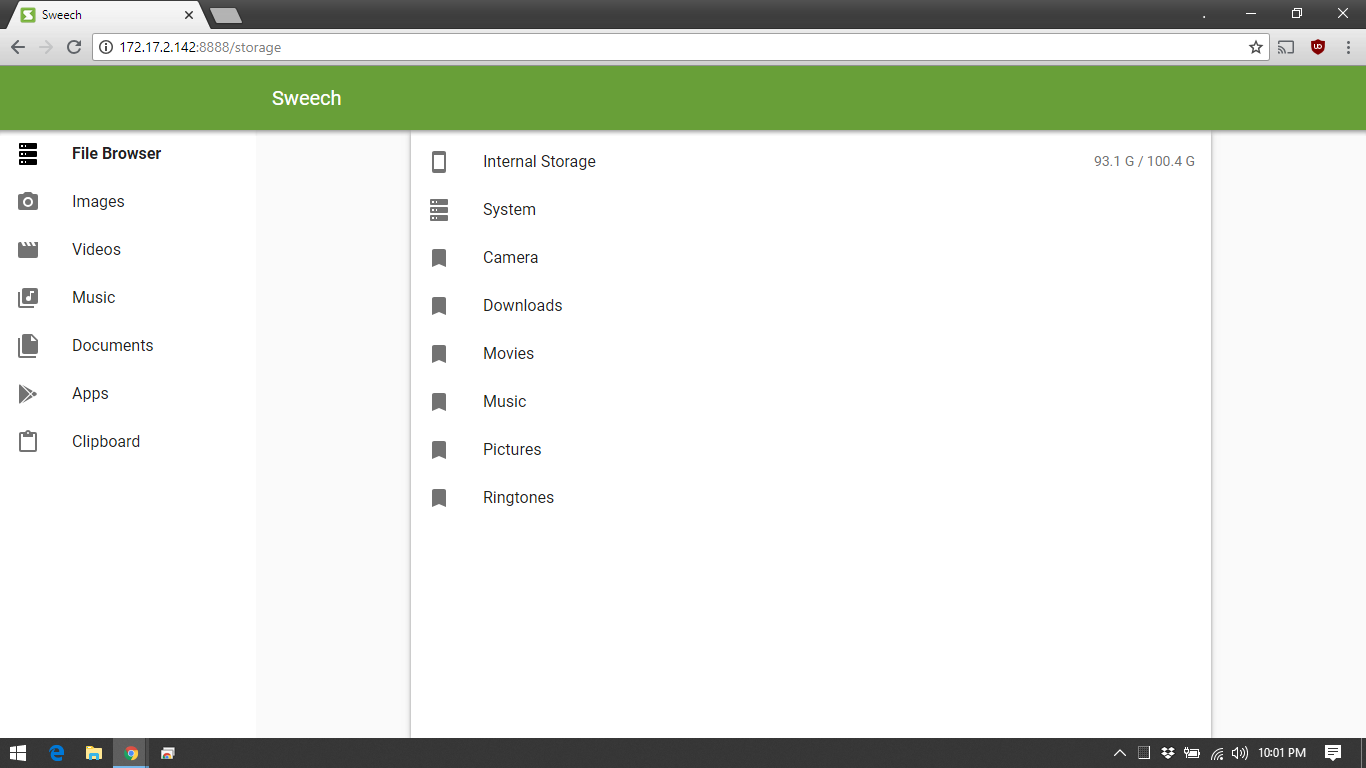The image displays a detailed view of a storage information screen on a Windows laptop. The taskbar, a dark grey strip at the bottom of the screen, indicates that it is a Windows operating system. From left to right, the taskbar includes the Windows Start button, Internet Explorer icon, File Explorer icon, Google Chrome icon, an unidentified network-related icon, and various system icons on the far right. These system icons include an upward-pointing arrow, a Dropbox icon, battery status, WiFi signal, sound settings, the time (10:01 PM), and a notifications icon.

At the top of the screen, a browser window is open, showing an IP address (172.17.2.142:8888/storage) in the address bar. The open tab displays "Sweesh," represented by a green square icon with a white squiggle inside, and the service name is spelled "S-W-E-E-S-H." Below the address bar, a green strip spans the width of the screen with the word "Switch" in white text.

The main content area is organized into several storage categories: file browser, images, videos, music, documents, apps, and clipboard. Additionally, an internal storage section shows 93.1 GB used out of a total 100.4 GB. Other listed storage sections include system camera, downloads, movies, music, pictures, and ringtones, suggesting a comprehensive cloud storage service.